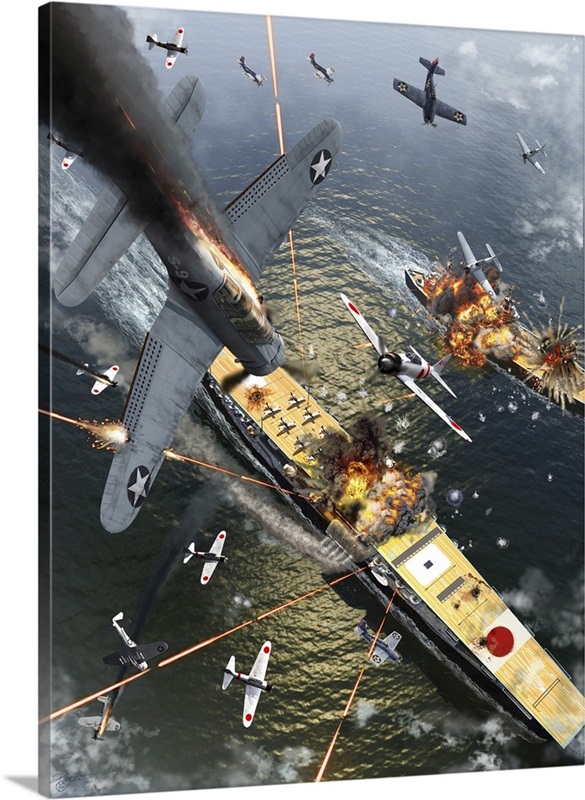This image is a highly detailed aerial view of an intense naval air battle in the ocean, vividly depicted on a wrapped canvas. Central to the scene is a large battleship diagonally oriented from the upper left to the lower right. The ship, with a red-topped deck, features the Chinese flag at its front. The middle of the ship is engulfed in an explosion, and we can see smaller planes stationed on its deck. Surrounding the central ship are numerous gray bomber planes marked with red dots, actively dive-bombing and attacking.

At the top left of the image, a plane with white stars on the underside of its wings is plummeting towards the water, trailing smoke and flames, indicating it has been shot down. Meanwhile, towards the top right, another smaller battleship is almost completely consumed by flames and smoke, under heavy attack.

Among the dramatic chaos, splashes in the water suggest bullets hitting the surface, adding to the fierce atmosphere of the battle. White planes with red dots and others with black circles and stars can be seen throughout the sky, orchestrating the assault. Adding to the intricate detailing, laser-like beams are fired from the ships below, further emphasizing the intensity of the combat on the high seas.